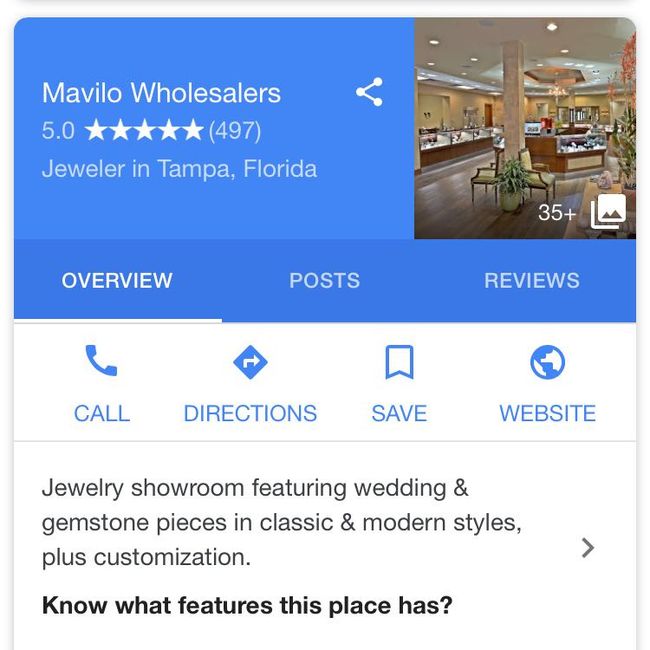The screenshot showcases a review of Malvalo Mavilo Wholesalers, a jewelry store located in Tampa, Florida. The store boasts an impressive rating of 5.0 out of 5.0, based on evaluations from 497 reviewers. The interface of the review includes an overview, posts, and reviews sections, all set against a sleek blue background. There is a small image depicting the storefront or interior of Malvalo Mavilo Wholesalers, adding a visual touch to the review.

Beneath this image, there are several interactive icons labeled "Call," "Directions," "Save," and "Website," each highlighted in blue. The text accompanying these icons describes the establishment as a "Jewelry showroom featuring wedding and gemstone pieces and classic modern styles, plus customization." This detailed description appears on a clean white background with black text, providing a clear and user-friendly interface.

The icons and labels "Call," "Directions," "Save," and "Website" are designed with blue accents, ensuring cohesive visual aesthetics. Additionally, a query at the end prompts users to explore the various features the store offers, inviting them to engage further with the business.